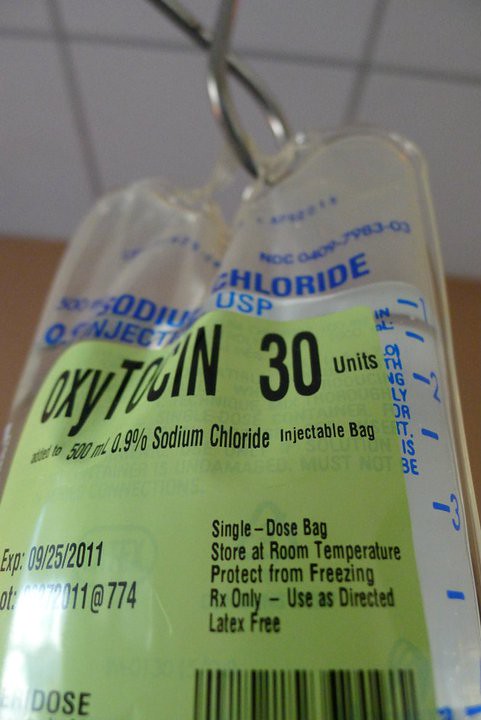The image depicts a clear IV bag commonly found in hospital settings, hanging from a metal apparatus. The bag contains 500 milliliters of 0.9% sodium chloride solution with an addition of 30 units of oxytocin. The label, marked with blue and green text, indicates it is an injectable bag with the expiry date of September 25, 2011. It is a single-dose bag, labeled "Rx only" and "latex free," with instructions to store at room temperature and protect from freezing. A barcode is present at the bottom of the bag, likely for scanning during use.